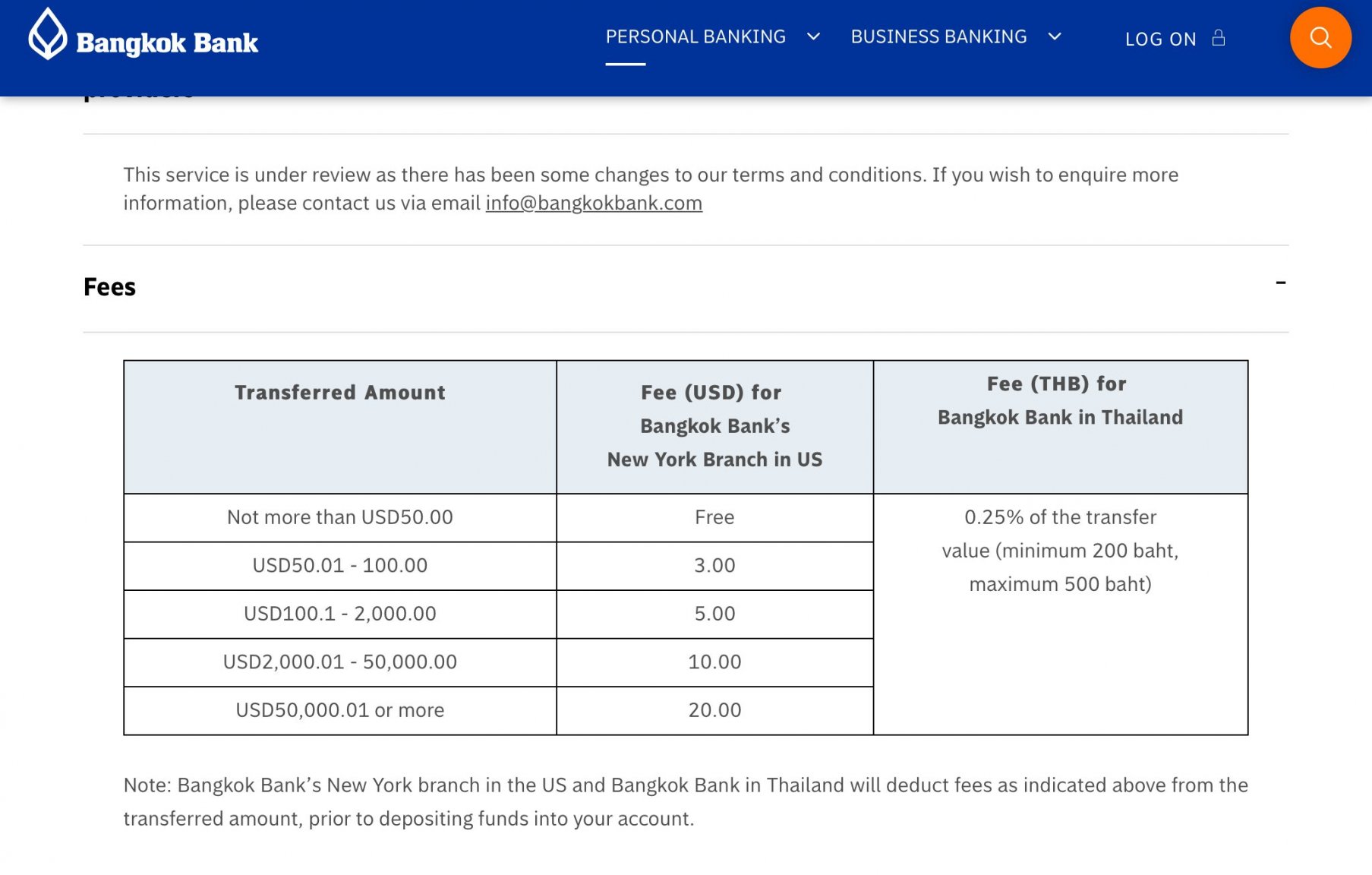### Caption

The image is a screen capture of a Bangkok Bank webpage. At the top, there is a navy-blue navigation bar with white text. Adjacent to the bank's name, "Bangkok Bank," is a leaf icon. The navigation bar includes several menu options: "Personal Banking," which is underlined in white, "Business Banking," each with a dropdown arrow, and "Log On," accompanied by a padlock icon. Beside the "Log On" section is an orange circle containing a white magnifying glass.

The main section of the webpage has a white background with black text. A notable message indicates that "The service is under review as there have been some changes to our terms and conditions. If you wish to inquire more about information, please contact us via email at info@bangkokbank.com."

Below the message, there is a detailed fee chart divided into three sections. The first section, highlighted with light blue at the top, details transfer fees in USD for Bangkok Bank's New York branch in the U.S.:

- Transfers not exceeding USD 50: free
- Transfers from USD 50.01 to 100: $3 branch fee
- Transfers from USD 100.01 to 2,000: $5 transfer fee
- Transfers from USD 2,000.01 to 50,000: $10 transfer fee
- Transfers of USD 50,000 and above: $20 transfer fee

The second section outlines the THB fees for Bangkok Bank in Thailand, specifying a flat fee of 0.25% of the transfer value, with a minimum of 200 baht and a maximum of 500 baht.

At the bottom of the chart, a note states, "Bangkok Bank's New York branch in the U.S. and Bangkok Bank in Thailand will deduct fees as indicated above the transferred amount prior to depositing funds into your account."